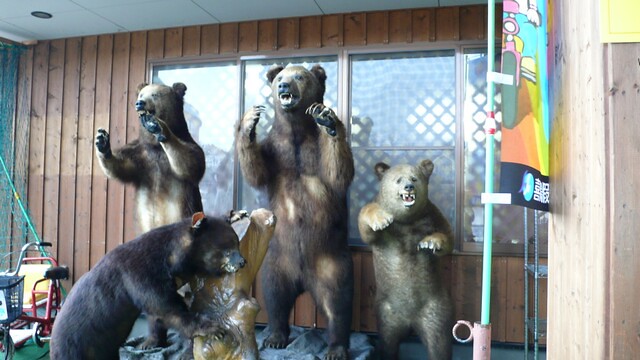This photograph captures four bear statues in front of an establishment accentuated by dark brown, timber wood panels. The bears exhibit a range of poses and fur colors, contributing to a dynamic and lifelike scene. Positioned near a blue-curtained window, the bears are crafted with meticulous detail. The three back bears, two of which stand tall around five feet, boast chocolate brown fur with tan and light brown accents. They have black noses, black eyes, and open mouths revealing pink tongues and teeth. A smaller bear on the right, roughly half the height of the tallest, displays a lighter brown fur interspersed with black splotches and similarly detailed facial features. 

In the foreground, another bear grips what appears to be a ceramic tree stump. This bear is black with pink details around its ears and light brown around its neck. Additional elements in the scene include a red tricycle with a basket on the left and a green net. A flag with Chinese writing and an illustration of a person riding a pink bicycle adds an international and playful touch to the rustic setting. These intricately detailed bears, combined with diverse props, create an intriguing and visually captivating display.